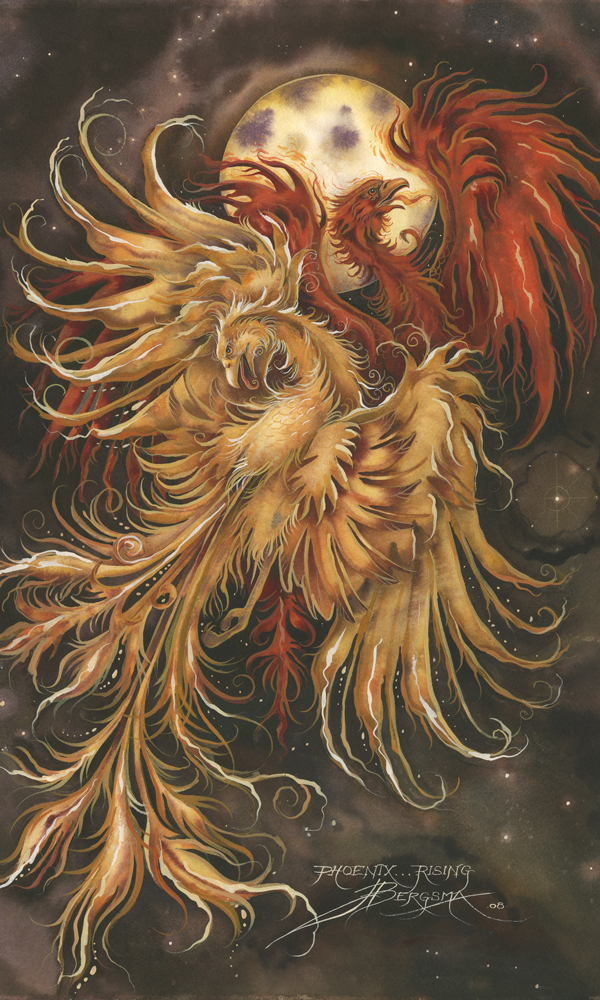The image showcases a vertical, colored painting dominated by two phoenixes, occupying about 70% of the picture. In the foreground, a golden phoenix with curly, wispy feathers is prominently displayed. Its long neck curves elegantly, and both its wings are spread out, with the right wing arched above and the left wing extended to the side. The phoenix's majestic tail feathers flow down towards the bottom left of the image. Behind it, a vibrant red phoenix, slightly obscured by the golden one, spreads its broad wings wide. This red phoenix’s head is slightly right of the golden phoenix and faces upward. The starry sky forms a dramatic backdrop, adorned with whitish-brown clouds and a glowing moon, yellow with gray spots. The moon is partially covered by the clouds and positioned just behind the red phoenix’s head. At the bottom of the painting, the text "Phoenix Rising Bergsma" can be seen, written in white.